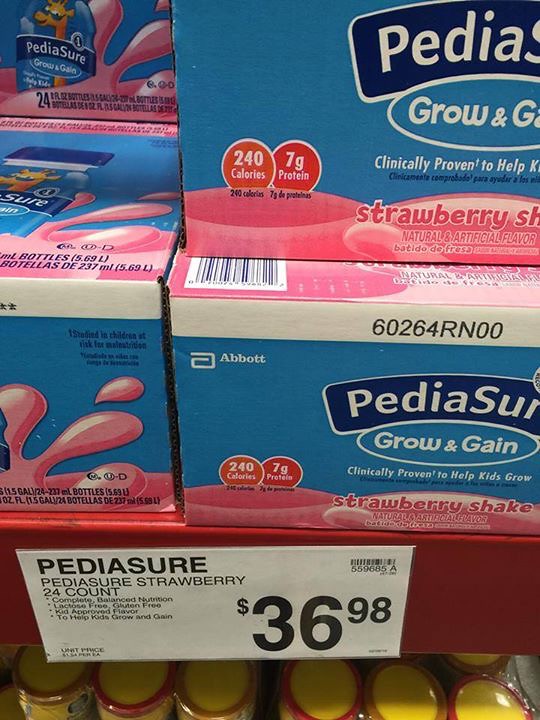The vertical, close-up color photograph captures stacked products of PediaSure Grow & Gain Strawberry Shake on a red metal shelf in what appears to be a bulk retail store. The horizontal, rectangular boxes are light blue with navy blue accents, prominently featuring the PediaSure logo in white font with the "P" and "S" capitalized. The label reads "Grow & Gain, Clinically Proven to Help Kids Grow" with additional details about being lactose-free and gluten-free. Each box includes nutritional highlights like "240 Calories" and "7g Protein" in red circles with white borders, partially visible due to the cropped image. Towards the bottom of the image, a white sign with black typeface in a clear covering states "PediaSure Strawberry, 24 Count" priced at $36.98. The photograph emphasizes the price and stacks of boxes against a backdrop of what appears to be yellow cans with red or gold rings in the lower section of the shelf.